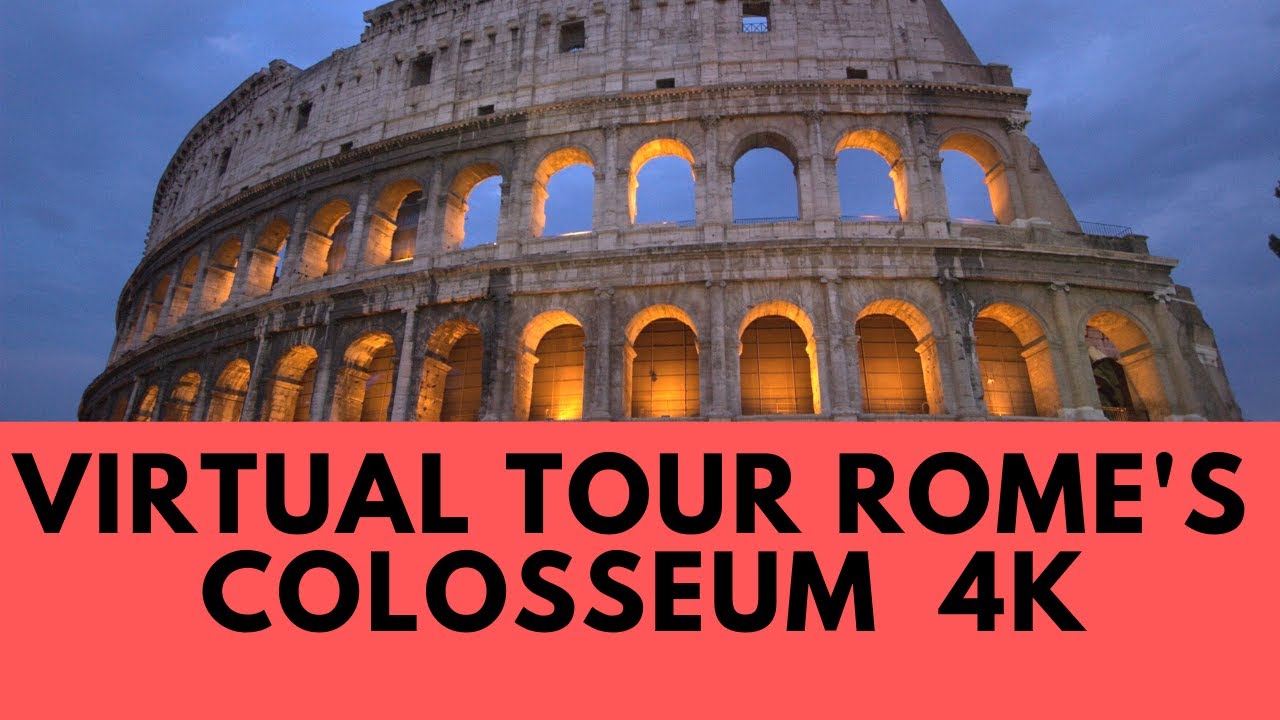The image is an advertisement for a virtual tour of the Roman Colosseum. The upper portion, which dominates the picture, displays the iconic structure at sunset against a dark blue, cloudy sky. The Colosseum is illuminated from within by warm, golden lights that permeate its arches, lending a glowing hue to its interior and upper levels. The topmost part of the Colosseum, previously characterized by jagged rocks, appears smoother and shows distinctive areas of ruin. A rectangular bar occupies the lower third of the image, featuring a muted pink background with bold, black, sans-serif text that reads in all caps: "VIRTUAL TOUR ROME'S COLOSSEUM 4K."